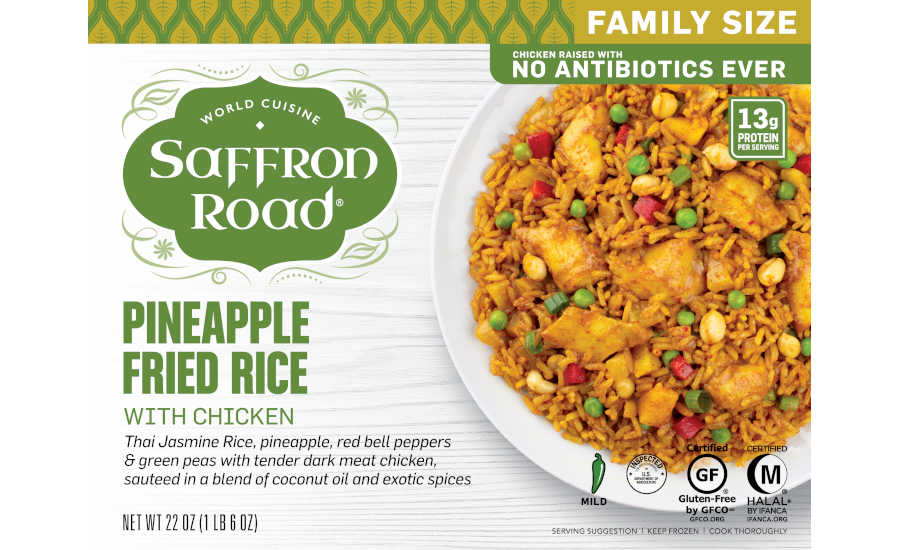This is an image of a family-sized box of World Cuisine Saffron Road Pineapple Fried Rice with Chicken. The box is predominantly white with green and gold trim, adorned at the top with an ornate "Saffron Road" logo, which includes a background of geometric patterns with leaves and swirly lines. Above this logo is "World Cuisine" in white text arced upwards, and a yellow and green leaf pattern stripe along the top edge of the box. In the upper right corner, it states "Family Size" in white text. Below that, it reads "Chicken Raised With No Antibiotics Ever" on a green background, followed by a badge indicating "13 grams of protein per serving."

The dish is described on the package as Pineapple Fried Rice with Chicken, featuring Thai Jasmine Rice, Pineapple, Red Bell Peppers, Green Peas, and tender dark meat chicken sautéed in a blend of coconut oil and exotic spices. The net weight is 22 ounces or 1 pound 6 ounces. 

A vibrant image of the dish occupies the center, showing a neatly presented plate of sautéed chicken, rice, peas, pineapple, and red bell peppers, suggesting a mildly spiced meal. Underneath the food image, there are four symbols: a green pepper indicating it has a mild spice level, a certification mark for Gluten-Free by the GFCO, and a Halal certification by IFANCA. The bottom of the package includes storage and preparation instructions: "Serving Suggestion: Keep Frozen. Cook Thoroughly." This well-detailed packaging makes it clear that the product caters to various dietary needs while offering an appetizing, exotic meal option for family dinners.